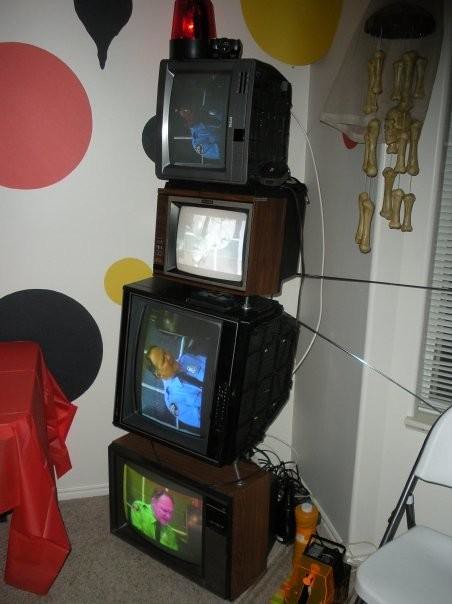In this vibrant color snapshot taken inside the corner of a room, likely within a house or apartment, four vintage tube televisions are intriguingly stacked atop one another, creating a quirky visual centerpiece. The bottom TV rests horizontally in a classic wood-imitating case with a black front, displaying a heavily magenta-hued image of what appears to be a policeman. The second TV, turned on its right side, corrects these colors, portraying the officer with more natural skin tones and a blue shirt. Above it sits a traditionally oriented black-and-white TV, while the top TV, tilted on its left side, shows a grayscale version of the same broadcast. Capping this peculiar tower is a red emergency strobe light, reminiscent of those found on police cars.

The visually stimulating backdrop features a wall festooned with large, colorful polka dots in shades of yellow, pink, red, and brown, and another wall painted in cream with a louvered window blind. To the left of the TV stack, a table draped in a red tablecloth adds more color to the scene, while a white plastic and metal folding chair sits in front of the window on the right. Completing this eclectic room are decorative elements, including hanging bones in the top right corner of the image, enhancing the eclectic and jumbled aesthetic of the space.